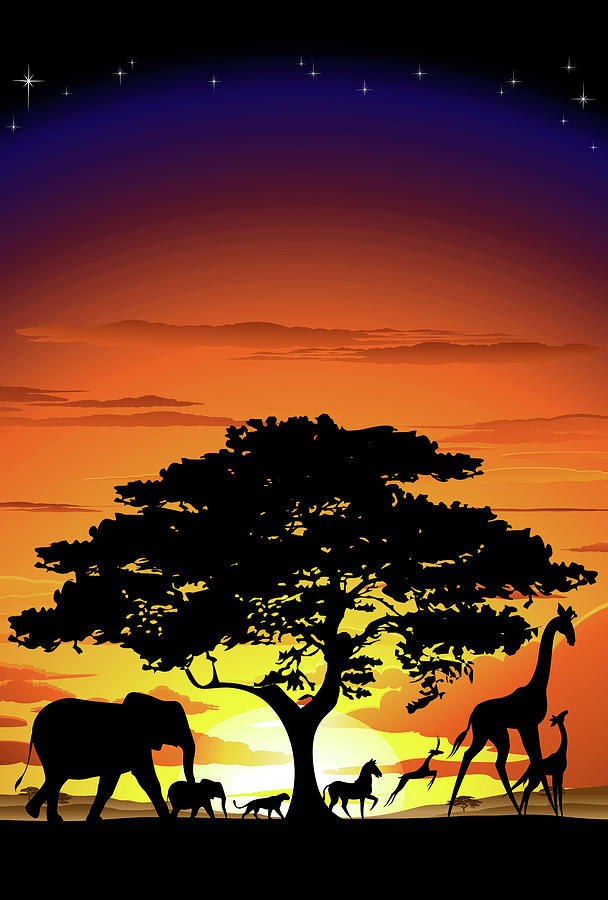This detailed graphic image depicts an enchanting outdoor night scene in a forest against a backdrop of either a sunrise or a sunset. At the top of the image, there is a dark blue sky sprinkled with twinkling stars, transitioning into a middle section featuring a dark orange sky adorned with gray or white clouds. Dominating the center is the silhouette of a broad, Y-shaped tree, its branches stretching from the left edge to the right edge of the image. The right side of the tree trunk is lush with leaves, while the left side has fewer.

In the bottom right corner, a captivating array of animal silhouettes brings life to the scene. First, two giraffes, a mother and her baby, appear to be walking with their shadows cast against the ground. Behind them stands a gazelle, followed closely by a horse with its front hoof raised in an elegant pose. Further back, a silhouette resembling either a leopard or a cheetah lurks, and behind that, the silhouettes of two elephants, one large and one smaller, complete the tableau. Every silhouette in this image is rendered in solid black, amplifying the striking contrast against the vibrant sky. The detailed and serene composition, devoid of any text, exudes a peaceful and enchanting atmosphere.